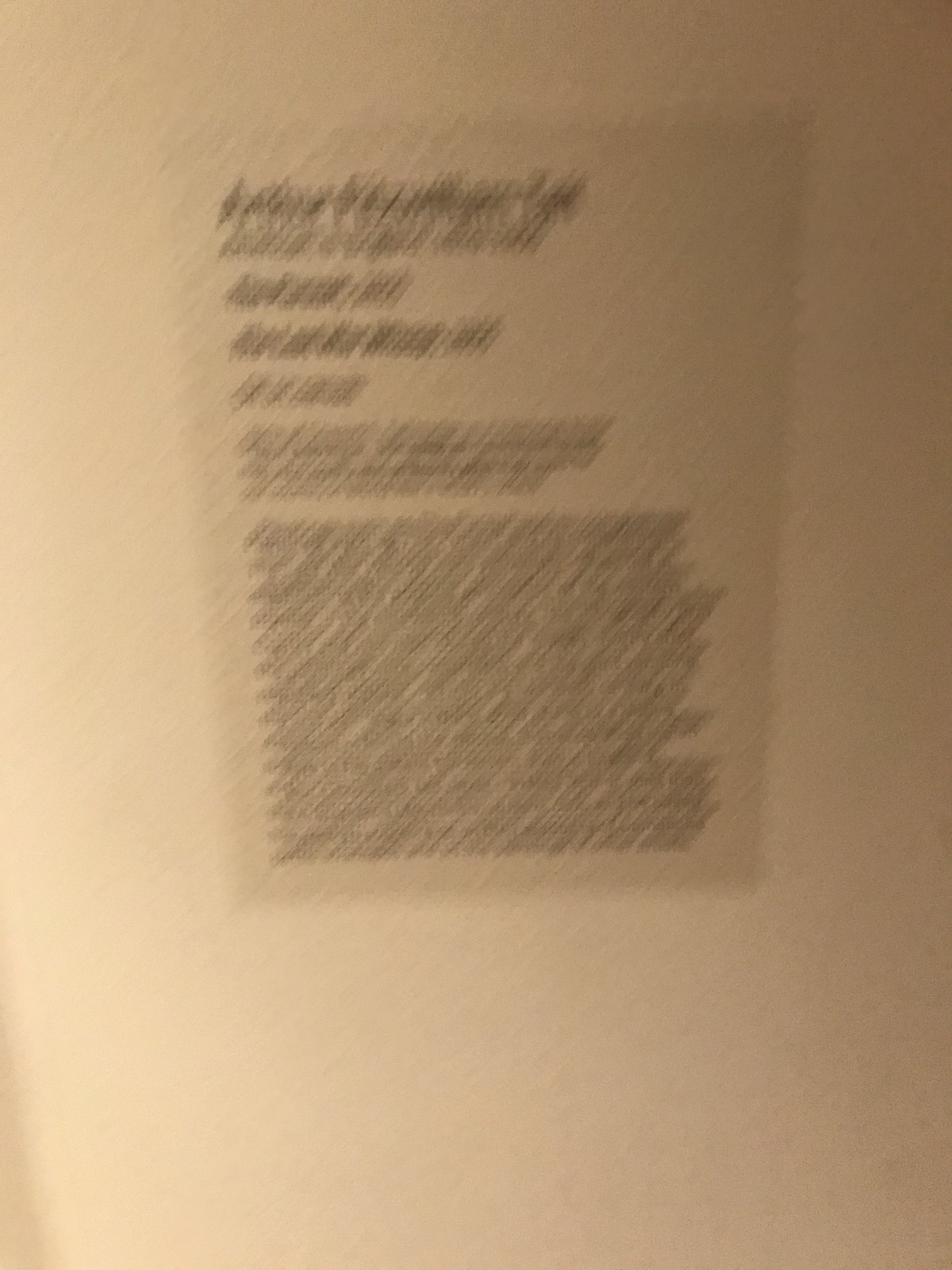The image features a photograph of a document set against a cream-colored background. The text in the document is blurred and entirely unreadable. At the top, the text begins in a larger, bold font, suggesting it might be a heading or title. Below the initial line, the font size decreases slightly with a secondary line that appears to have a similar number of characters. Following this, the text size diminishes even further, likely representing a subheading. The majority of the document consists of a dense block of text, estimated to be around 25 sentences in length, stretching from the middle of the page to the bottom. Despite the clarity issues, the document features uniformly black text.